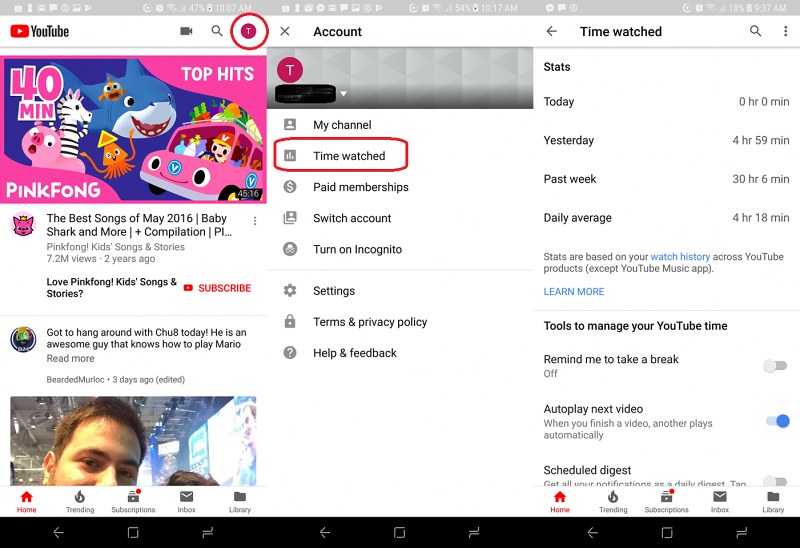### Detailed Caption of Android YouTube Screenshots

This image showcases a collage of three adjacent screenshots taken on an Android cell phone, each portraying various aspects of the YouTube app.

1. **First Screenshot (Left Panel):**
   - The topmost part features a standard Android status bar with battery power indicator, Wi-Fi signal strength, and other common icons.
   - Just below the status bar, the YouTube interface is visible with the recognizable YouTube logo and the search bar.
   - The primary focus is on a video titled "40 Minute Pinkfong Top Hits," indicating a collection of kids' songs and stories. Beneath this, another video is partially visible with the title "Got to hang around with Chewate today. He is an awesome guy that I've known to play Mario."
   - A small thumbnail image of a person’s face appears at the lower part of this panel.
   - At the bottom, the navigational bar provides options to browse Home, Trending, Subscriptions, Inbox, and Library.
   - The lowest section displays the Android navigation options such as back, home, and recent apps.

2. **Second Screenshot (Middle Panel):**
   - This panel begins with the account section indicated by the word "Account" at the top.
   - Below the header, the user’s profile icon is displayed followed by several menu items including My Channel, Time Watched, Paid Memberships, Switch Account, Turn on Incognito, Settings, Terms and Privacy Policy, and Help and Feedback.
   - Highlighted in this screenshot, the "Time Watched" option is encircled, drawing attention to its selection.

3. **Third Screenshot (Right Panel):**
   - The final panel dives deeper into the "Time Watched" statistics screen.
   - It presents a summary of YouTube usage with categories like Today, Yesterday, Past Week, and Daily Average.
   - Additionally, it lists "Tools to Manage Your YouTube Time," featuring options such as Remind me to take a break, Autoplay next video, and Schedule digest.
   - This panel serves as a practical guide on setting viewing limits, offering tools and statistics to help manage and monitor YouTube watch time, beneficial for both personal use and parental control.

The collective presentation of these screenshots appears to form a tutorial aimed at educating users on how to set and manage viewing limits on YouTube, emphasizing user responsibility and time management.